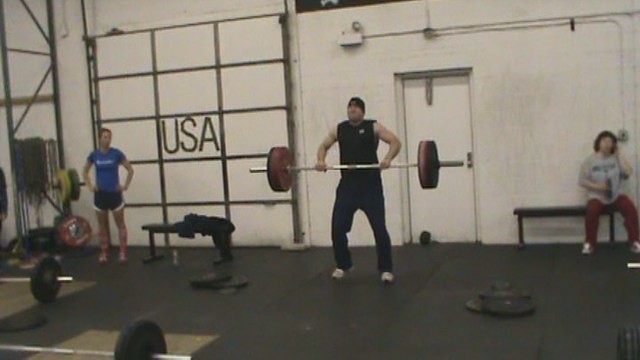The image captures an old-school gym setup with black rubber mats covering the floor and white-painted walls. Dominating the scene is a muscular individual in the center, wearing a black sleeveless shirt, black pants, a black knit hat or backwards baseball cap, and white shoes. They are lifting a curling bar loaded with both red and black weights. To the left, a toned woman with short brown hair is dressed in a blue t-shirt with blurred white writing, dark blue shorts with white accents, and pink-and-white shoes or boots. She stands near a barbell with yellow and dark green weights, amid scattered exercise bands and loose weights. On the right, another person with short curly brown hair is seated on a black bench with wooden legs, dressed in a gray shirt with dark blue text, long red pants, and white shoes with accents. They appear to be holding a bottle. The backdrop features a distinct 'USA' sign within a grid pattern, seemingly crafted from tape, positioned near a door with a push bar. The overall ambiance of the gym is minimalist, emphasizing free weights and benches over modern gym machines.